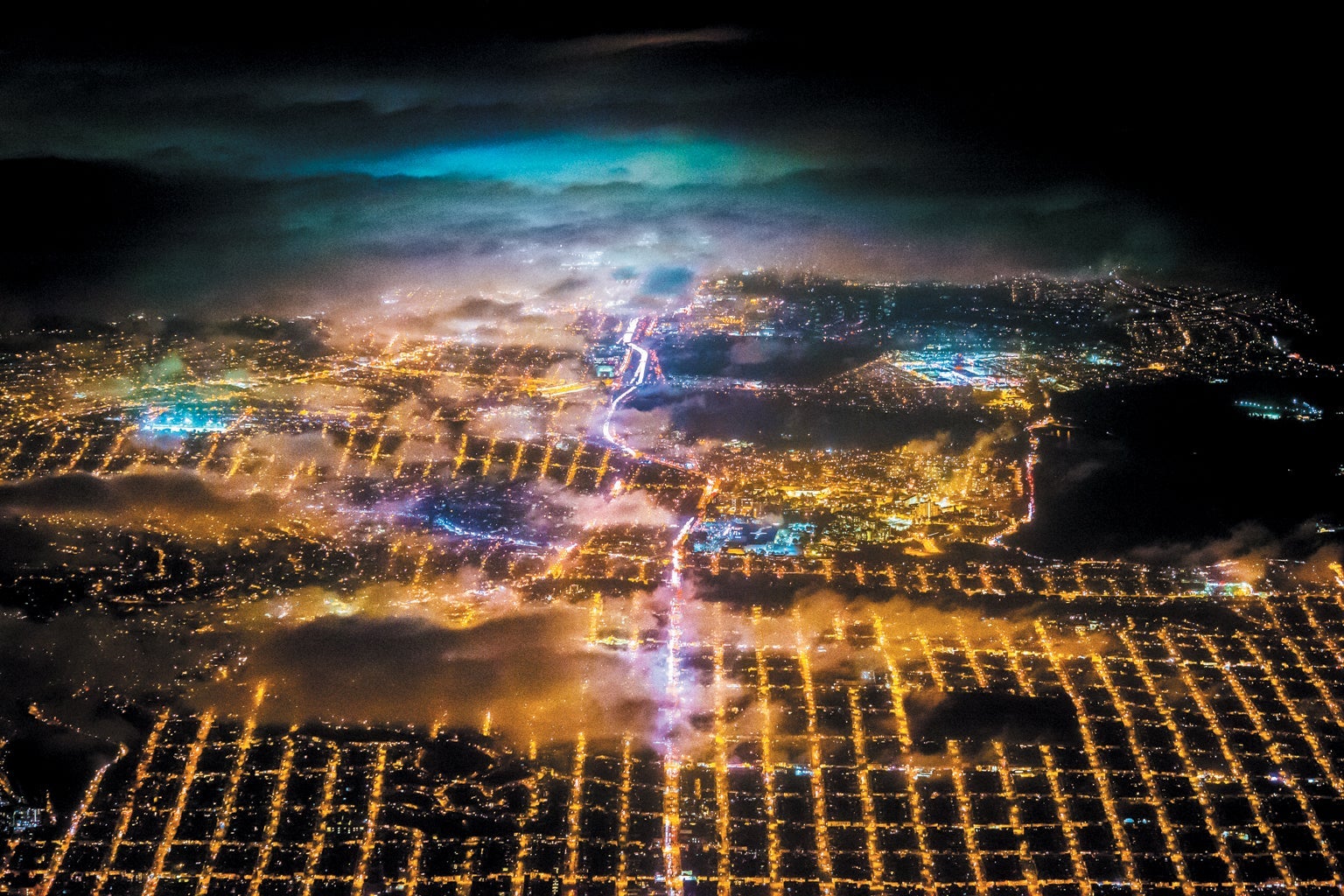This image is an aerial nighttime view of a city, blending realism with surrealistic elements, possibly computer-generated or heavily edited. The lower half of the image features a yellow to light orange grid overlaying the city, illuminating the structures beneath with an intense, almost artificial glow. This grid slightly breaks apart as it extends into the middle of the image, where a distinct beam of light travels vertically, dividing the cityscape from the bottom all the way to the top of the frame. 

In the darker regions, presumed to be bodies of water, there are no lights, providing a stark contrast to the brightness of the city's buildings. There are clouds both above and below the viewer: the lower clouds are illuminated by the city's lights, while the higher clouds remain largely dark, except for a distinct turquoise area in the center that brightens the scene uniquely. 

In the background, the color palette transitions to more fluorescent tones, culminating in a bright, neon blue sky, inconsistent with the expected darkness of nighttime, adding to the image's surreal quality. The abundance of lights, coupled with the grid overlay and unusual sky color, gives the entire scene a dreamlike, otherworldly atmosphere, reminiscent of scenes from video games or digitally enhanced artwork.